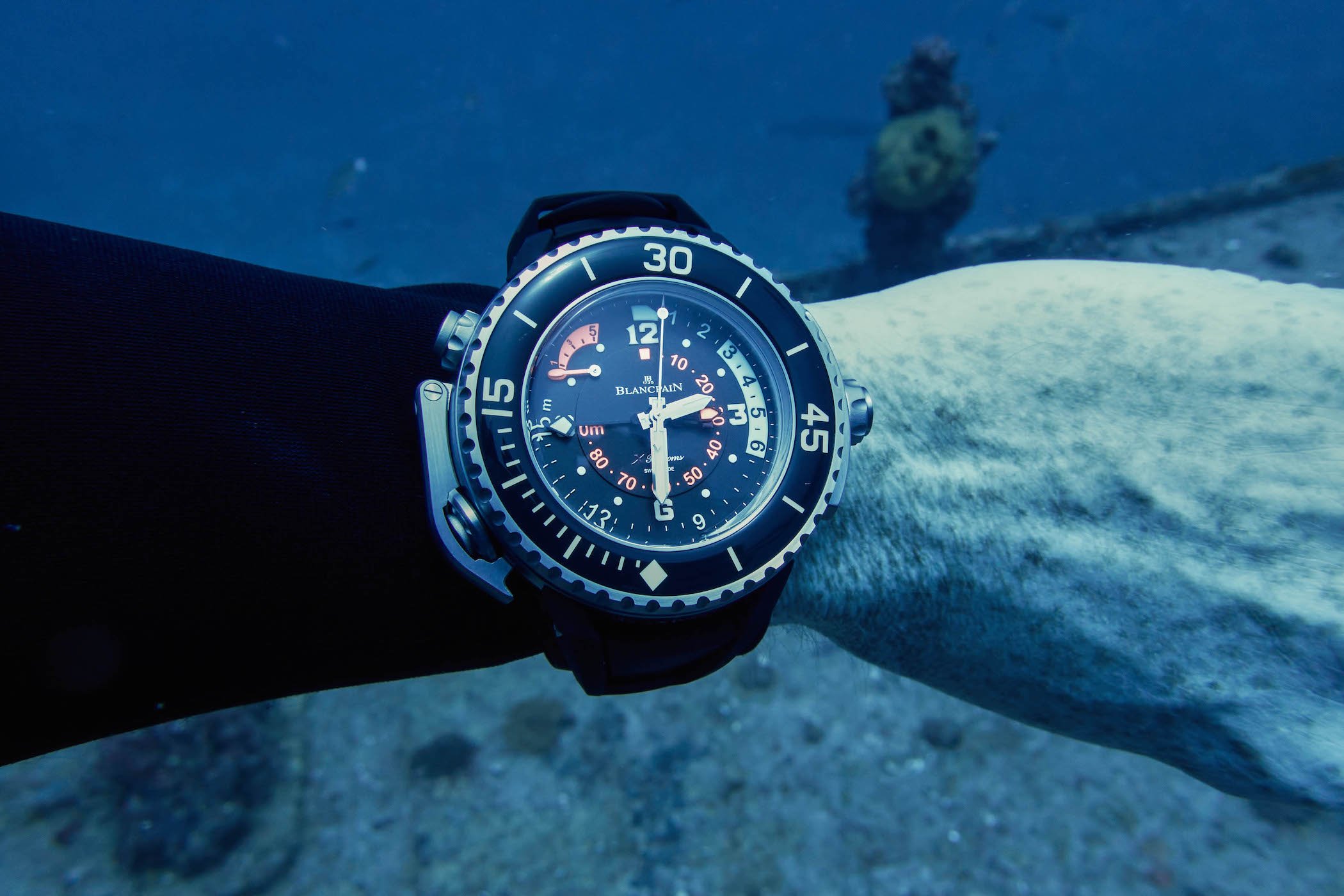The image showcases a close-up of an older diver's wrist, clad in a black scuba suit, set against the backdrop of the ocean floor. The central focus is on a large, specialized diver's watch with a dark blue or black face, complemented by silver trimmings, making it easy to read underwater. The dial features white and salmon-colored numbers and includes an adjustable outer ring with 0, 15, 30, and 45-minute markings, likely used for timing dives or measuring remaining air supply. The diver's hand, with visible skin spots and aging lines from sun exposure, adds depth to the underwater scene. The background hints at an old shipwreck amidst the water's blue hue, devoid of coral or fish. The watch appears durable and expensive, designed to withstand underwater pressure, and prominently displays its brand at the center.